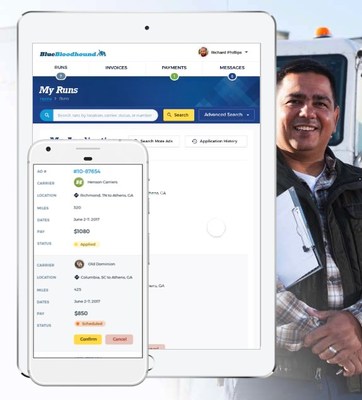In a partially obscured background, a man with tan skin is standing inside a truck, exuding a confident and friendly demeanor. He has short, dark hair and is gazing directly at the camera with a wide smile. Dressed in a dark-colored jacket layered over a long-sleeved plaid shirt, he holds a clipboard securely under his right arm. His hands are clasped in front of him, and a wedding ring is visible on his left hand. To the left side of the image, a tablet is displayed, featuring a blue banner with the partially legible phrase "My Runs" and a visible search bar. Positioned above the tablet is a cell phone with indistinct writing on its screen. The scene contains no animals, plants, flowers, trees, motorcycles, bicycles, or airplanes.